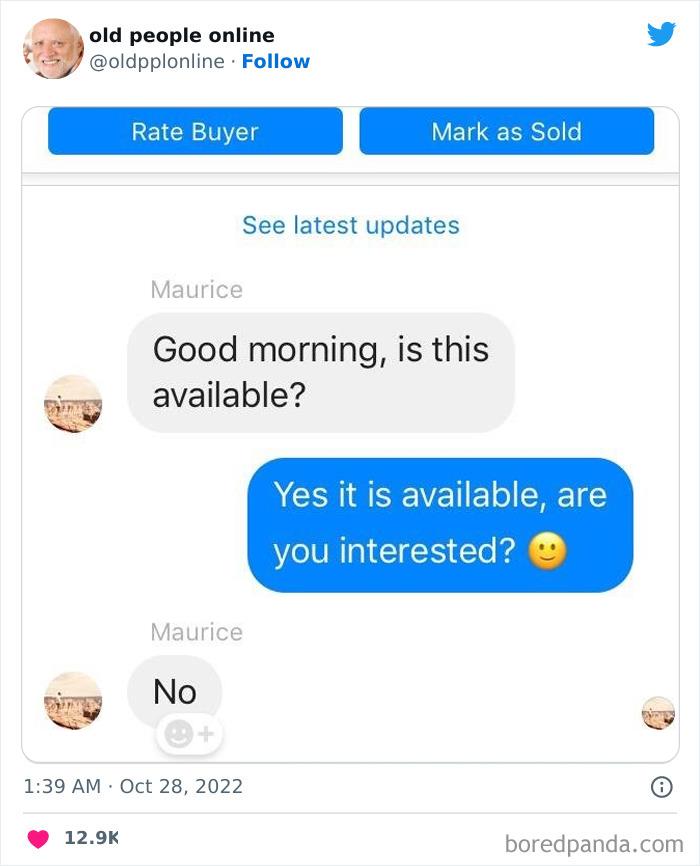Screenshot from a website on a white background featuring a humorous Twitter post. At the top, there's a picture of an older man smiling, with the text "Old People Online" beside it, indicating the account name, followed by a "Follow" button. A blue Twitter bird icon is situated in the upper right corner. Below, two blue buttons read "Rate," "Buyer," "Mark," and a green "Sold."

In the center, a grey text box displays the conversation:
- Morris: "Good morning, is this available?" (next to a small beach photo icon)
- Response: "Yes, it is available, are you interested?"
- Morris: "No."

The timestamp indicates the conversation took place at 1:39 AM on October 28th, 2022. Below this, on the left, there are 12.9k likes accompanied by a heart icon. In the lower right, a watermark indicates the post is from boredpanda.com. 

The content humorously parodies older individuals online as being awkward and disinterested, hinting at ageist stereotypes yet evoking a sense of comedic irony.